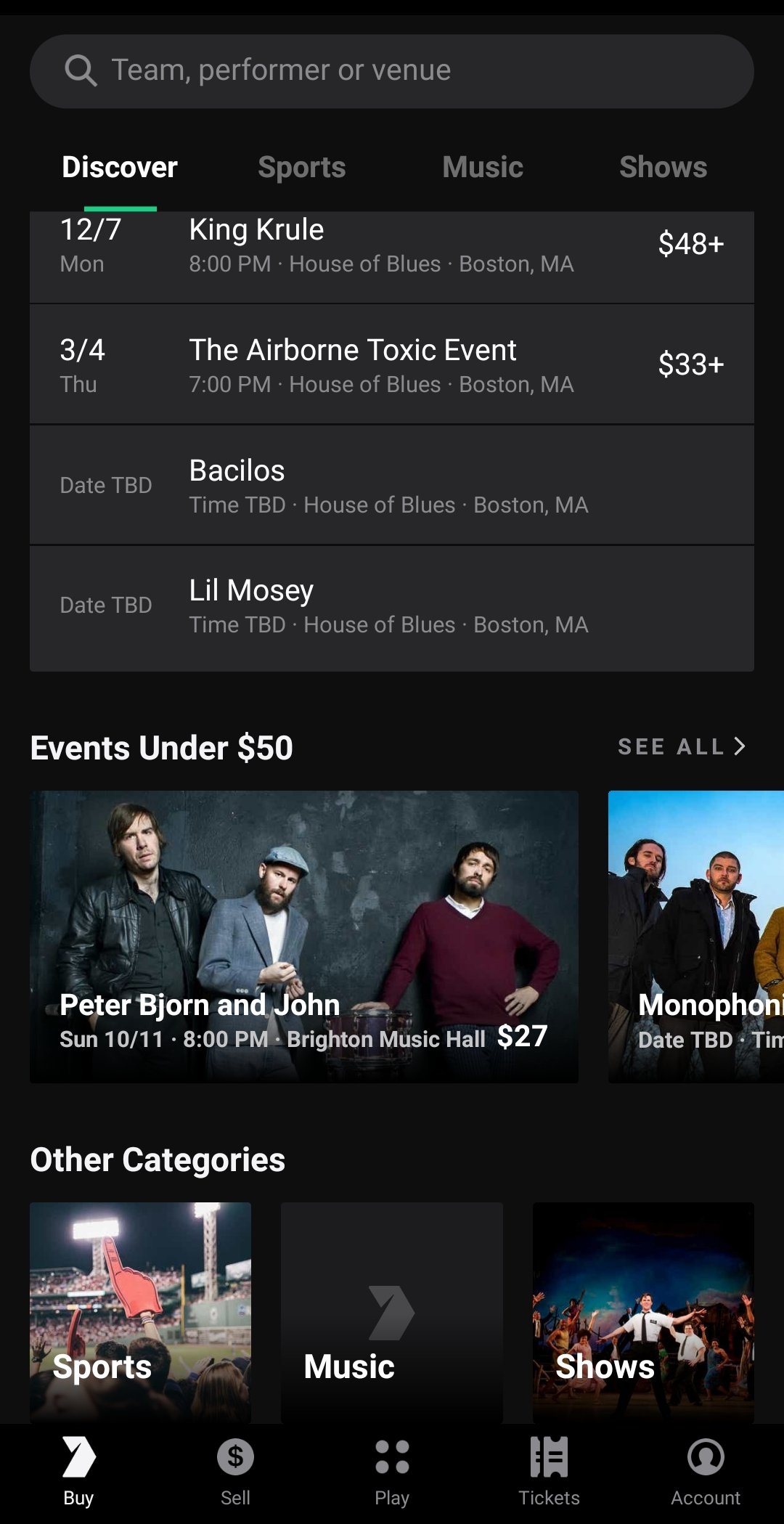This image showcases a mobile app interface designed for buying and selling tickets for various events, including concerts and shows. At the top of the interface, there is a search bar labeled "Search team, performer, venue," allowing users to find specific events. Below the search bar, the interface is organized into four main tabs: "Discover," "Sports," "Music," and "Shows." 

The "Discover" tab displays a list of upcoming events, starting with a concert by King Krule at the House of Blues in Boston, Massachusetts, priced at $48. Another listed event is The Airborne Toxic Event, also at the House of Blues, priced at $33. 

Scrolling further down, users can find events categorized under a budget-friendly section titled "Events Under $50," which includes a concert by Peter Bjorn and John at Brighton Music Hall, with tickets available for $27. 

As users navigate further, events are segmented into specific categories like "Sports," "Music," and "Shows," making it easier to find events of interest. At the bottom of the app, five main subsections are visible: "Buy," "Sell," "Play," "Tickets," and "Account." The "Play" section remains unclear, but the app appears to also offer features for event listing and management.